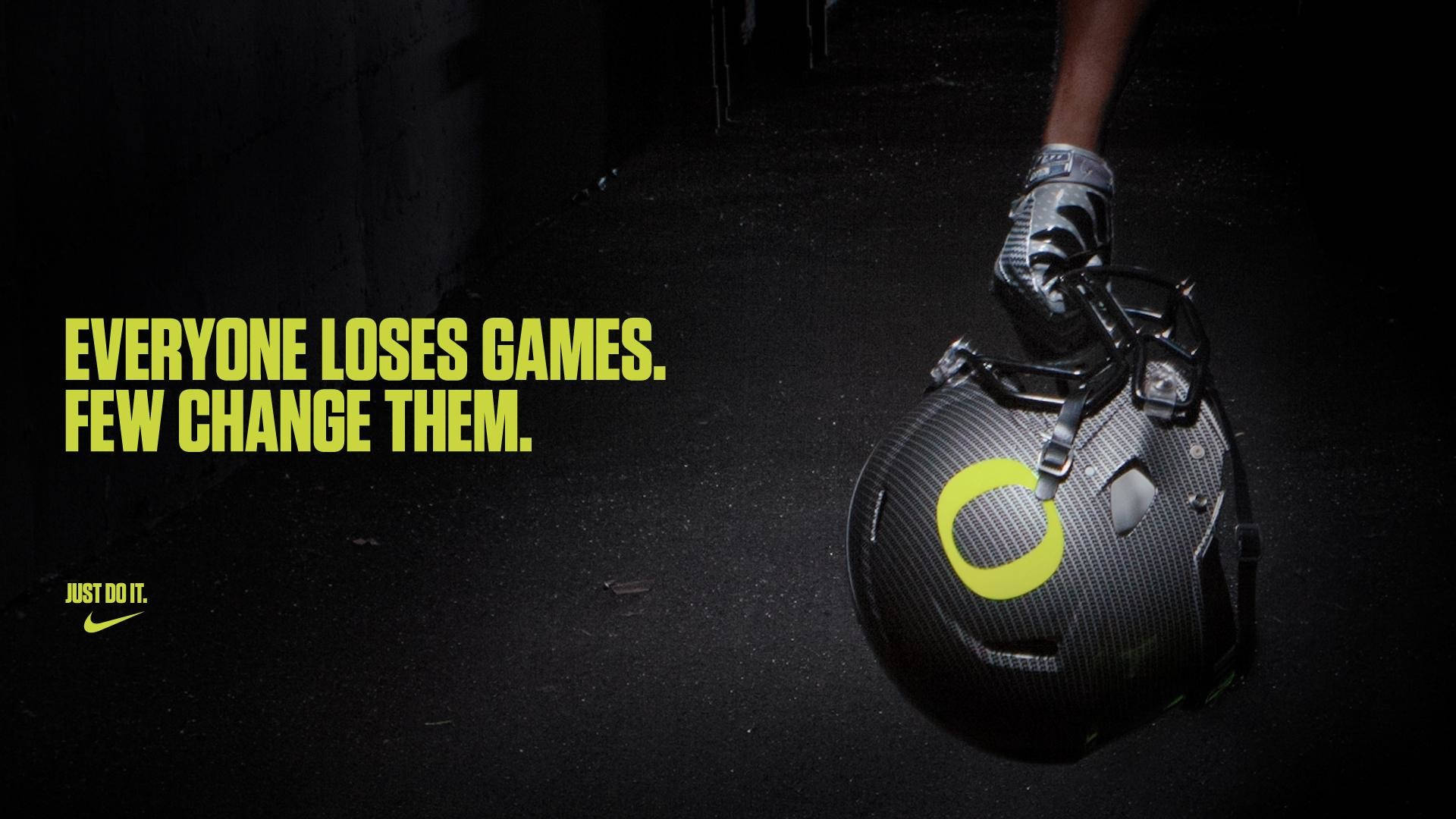The Nike print advertisement features a predominantly black background with a slight grainy texture. On the left side, bold yellow text reads, "Everyone Loses Games. Few Change Them." Below this tagline is the iconic Nike logo with the phrase "Just Do It" and the signature Nike swoosh. On the right side, emerging from the top-right corner, is a gloved hand clad in a silver glove with black decals, grasping a football helmet. The helmet, designed with black, gray, and white stripes and a black face mask, prominently displays a yellow "O" on its side. The entire image is framed by a subtle white haze, highlighting the football helmet and the gloved hand against the dark background.